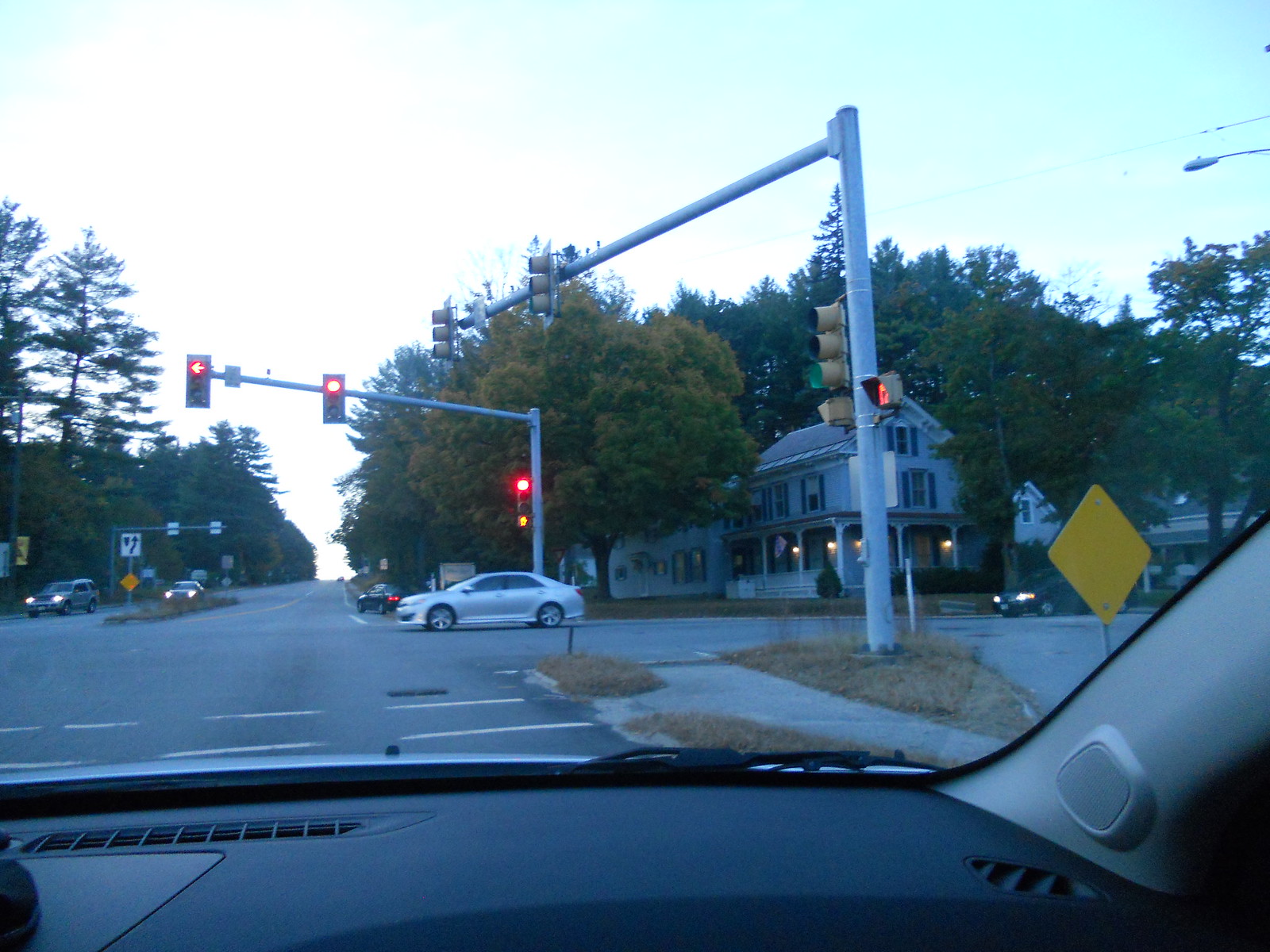A vivid photograph captured from inside a car, through the front windshield, depicts a moment paused at a red light. The glaring red traffic signal commands attention in the center of the frame, confirming the vehicle's halted state. To the right, a car is in the midst of entering the intersection, just beginning its journey across. Adjacent to this car is an empty sidewalk and crosswalk, devoid of pedestrians. Inside the vehicle, the top of the dashboard is visible, along with an air vent. A streetlight pole extends upwards from the right side of the frame. Across the street stands a striking Victorian-style white house, enclosed by a pristine white fence, adding a touch of historic elegance to the scene.